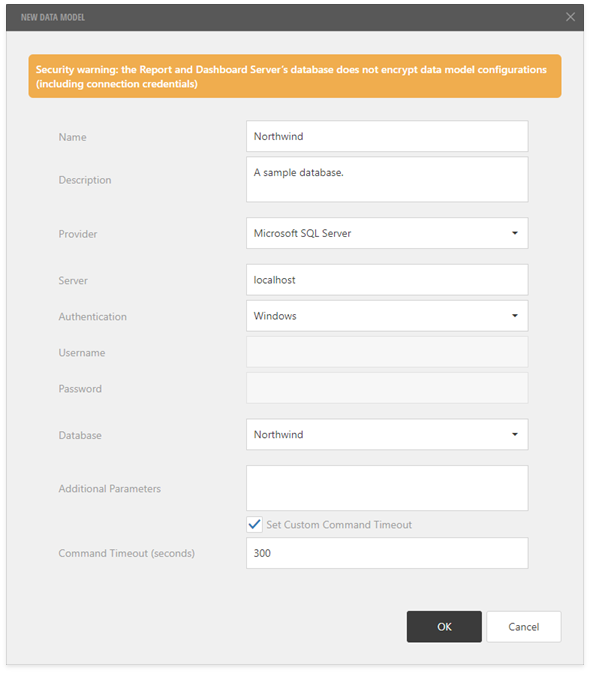This image depicts a user interface with a predominantly gray background and a black horizontal bar at the top. In the upper left corner of the bar, in uppercase gray text, it reads "NEW DATA MODEL." In the upper right corner, there's a gray "X" indicating an option to close the window.

Beneath the top bar, approximately three lines down and center-aligned against the gray background, is a conspicuous orange rectangle. Below this rectangle, the interface is laid out in a form-like structure.

The form begins with a series of labels and corresponding input fields:
1. **Name:** On the left in gray text, with an adjacent white text box on the right for the user to input the name.
2. **Description:** Similar setup as Name, with a white text box provided for user input.
3. **Provider:** This is a dropdown menu displaying "Microsoft SQL Server" in black text.
4. **Server:** A labeled input field where "localhost" is pre-filled within the white text box.
5. **Authentication:** Another dropdown menu with "Windows" currently selected.

Following these fields are:
6. **Username and Password:** Both are presented with gray text boxes intended for user input.
7. **Database:** A dropdown menu indicating "Northwind" is selected.
8. **Additional Parameters:** Beneath this label is a white text box for more details. Below this box, there's a white checkbox with a blue checkmark next to the option labeled in gray text, "Set custom command timeout."
9. **Command Timeout (seconds):** This field has a white text box pre-filled with the value "300."

At the lower right corner of the interface, there are two buttons. The left button is black and labeled "OK," while the right button is white and labeled "Cancel."